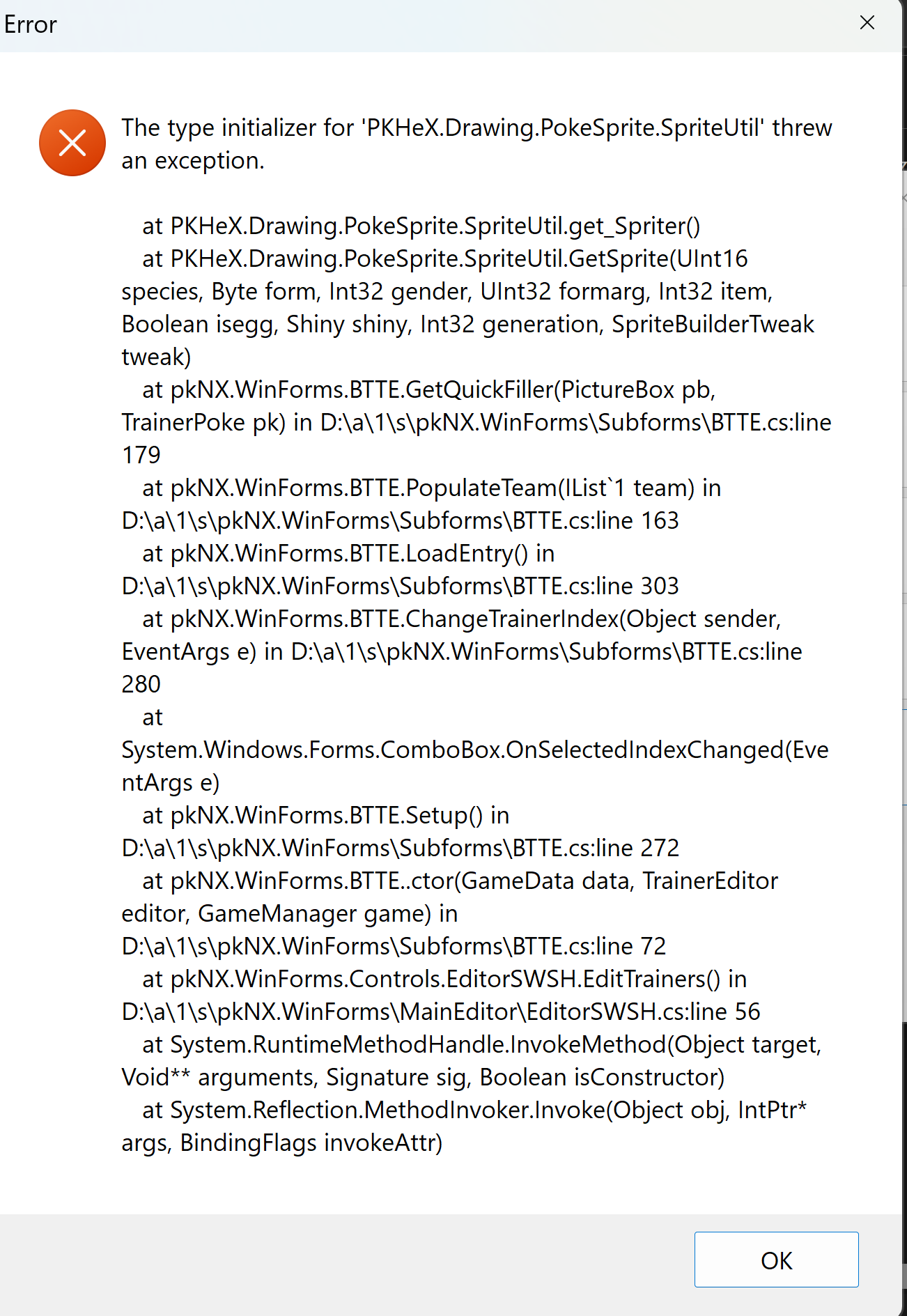This image is a detailed vertical screenshot, primarily displaying an error pop-up box against a white backdrop. At the top and bottom of the image, there are thin light gray lines serving as banners. 

In the top-left corner, the pop-up is labeled as an error in black typeset. The pop-up content begins with a gray horizontal strip, just beneath which there is a striking orange-red circle with a white "X" through it, signifying an error. 

The text following this symbol indicates a specific type of error: "The type initializer for pkhex.drawing.pokesprite.spriteutil threw an exception." 

Below this message, there are numerous lines of black text written in coding language, which provide a detailed account of the error. The first line reads: "at pkhex.drawing.pokesprite.spriteutil.get_spriter()". This is followed by what appears to be between 40 to 50 lines of additional code, offering a comprehensive description of the error encountered.

At the bottom right corner of the pop-up, enclosed within a thin blue border, is a horizontally-oriented rectangular button that reads "OK". This button allows the user to acknowledge the error message and close the pop-up.